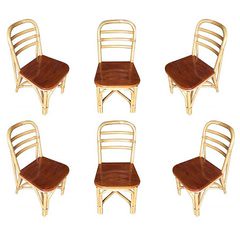The illustration features six small chairs, appearing possibly as dollhouse furniture, arranged against a plain white background. They are systematically organized into two rows of three chairs each. Each chair has a metallic, gold-colored frame with an upside-down U-shaped backrest, which includes three horizontal bars. The legs of the chairs curve inward, forming an X-shaped support underneath, and the seats are a medium brown wood with a glossy finish. The seating area and the top of each chair are square and dark brown.

The chairs are depicted at different angles, creating a mirrored arrangement between the two rows. In both rows, the left chair faces diagonally to the right, the middle chair is viewed from the front, and the right chair faces diagonally to the left. 

This detailed layout presents a downward perspective, almost as if looking from an angle in the upper corner of a room, providing a comprehensive overview of each chair’s design and orientation.